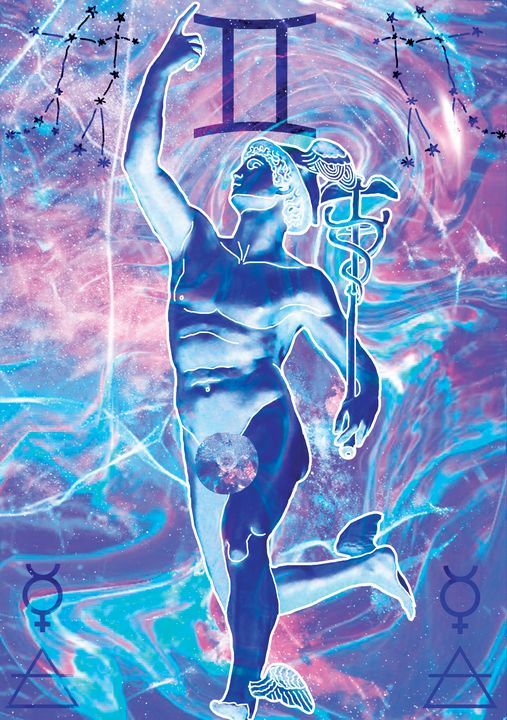In the center of the image stands a computer-generated depiction of an ancient Greek-like statue, closely resembling the god Mercury, identified by the wings on its ankles. The statue, holding a staff resembling the caduceus—a symbol for medicine—features a blue snake coiled around the staff. This figure points upward with its right hand towards the Gemini symbol positioned above its head, indicated by the Roman numeral II. The background of the image is a galaxy-like swirl of vivid colors including purple, blue, magenta, pink, and various other hues. Constellations, appearing as human figures holding hands, adorn the top left and right corners of the image. At the statue's feet, there are two female gender symbols located on either side, each placed above a triangle with a horizontal line crossing through it. The statue itself, likely representing Mercury, orbits within a scene both mystical and celestial, combining elements of mythology with the expansive beauty of the cosmos.